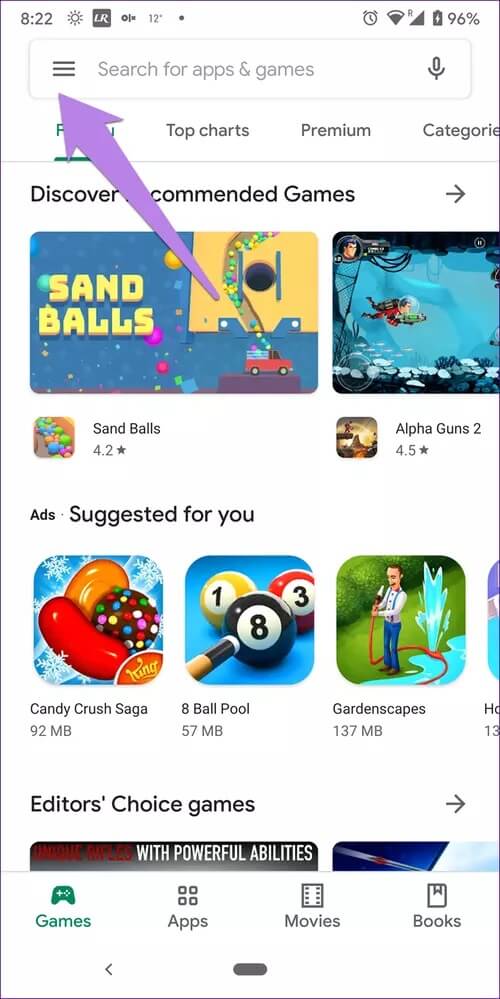A detailed smartphone screenshot displays various elements characteristic of a weather and app store interface. At the top, the status bar shows the current time accompanied by a sun icon, suggesting daytime. Nearby, a gray square with white letters "UR" is visible alongside a weather indicator showing "12°" within a black circle. Adjacent are icons symbolizing signal strength, a power signal, a triangle, and a battery at 96%.

Below the status bar, a gray-bordered search bar with three black lines displays "Search for apps and games" in gray capital letters and includes a microphone icon. Immediately beneath, a purple arrow points to three bars obscuring part of the first of four subcategory titles in green lettering. The remaining titles are "Top Charts," "Premium," and "Categories," all in bold capital letters. Separating them, a thin gray line underscores the green text.

Further down, a prominent section titled "Discover Comended Games" (with a spelling error) is highlighted with a right-facing gray arrow. This section features two cartoonish image previews. The first image, under the title "Sandballs," has bold yellow letters on a blue background filled with colorful balls in red, purple, green, and yellow. A toy truck at the bottom, with a red body and yellow "M," is depicted amid floating balloons. Beside it, another image portrays an underwater scene with a character wearing a red snorkeling outfit and surrounded by sea elements and bubbles. A small square in the corner shows a cartoon face, reinforcing the aquatic theme.

Below these images, "Sandballs" is reiterated in black letters next to a rating of 4.2 and a black star. Adjacent, an unclear image with a yellow background, possibly a lighthouse, is labeled "Alpha Guns" with a rating of 4.5 and a black star. Below these descriptions, the section title "ADS: Suggested for You" introduces three recommended games: "Candy Crush Saga" (92 MB), illustrated with candy-like elements; "8 Ball Pool" (57 MB), showcasing billiard balls and a cue stick; and "Gardenscapes" (137 MB), featuring a man using a red hose next to a river, with a playful water spray.

Deeper in the layout, an "Editor's Choice Games" segment marked by a gray bar highlights "Powerful Abilities" in white letters. To its right, a green icon resembling a game controller and a green "Games" label delineate the area. Nearby, four black circles under "Apps" and a black square with side dots labeled "Movies" formalize additional categories. Lastly, a gray rectangular "Books" section with a rounded button concludes the capture, symbolizing easy access to book-related media.